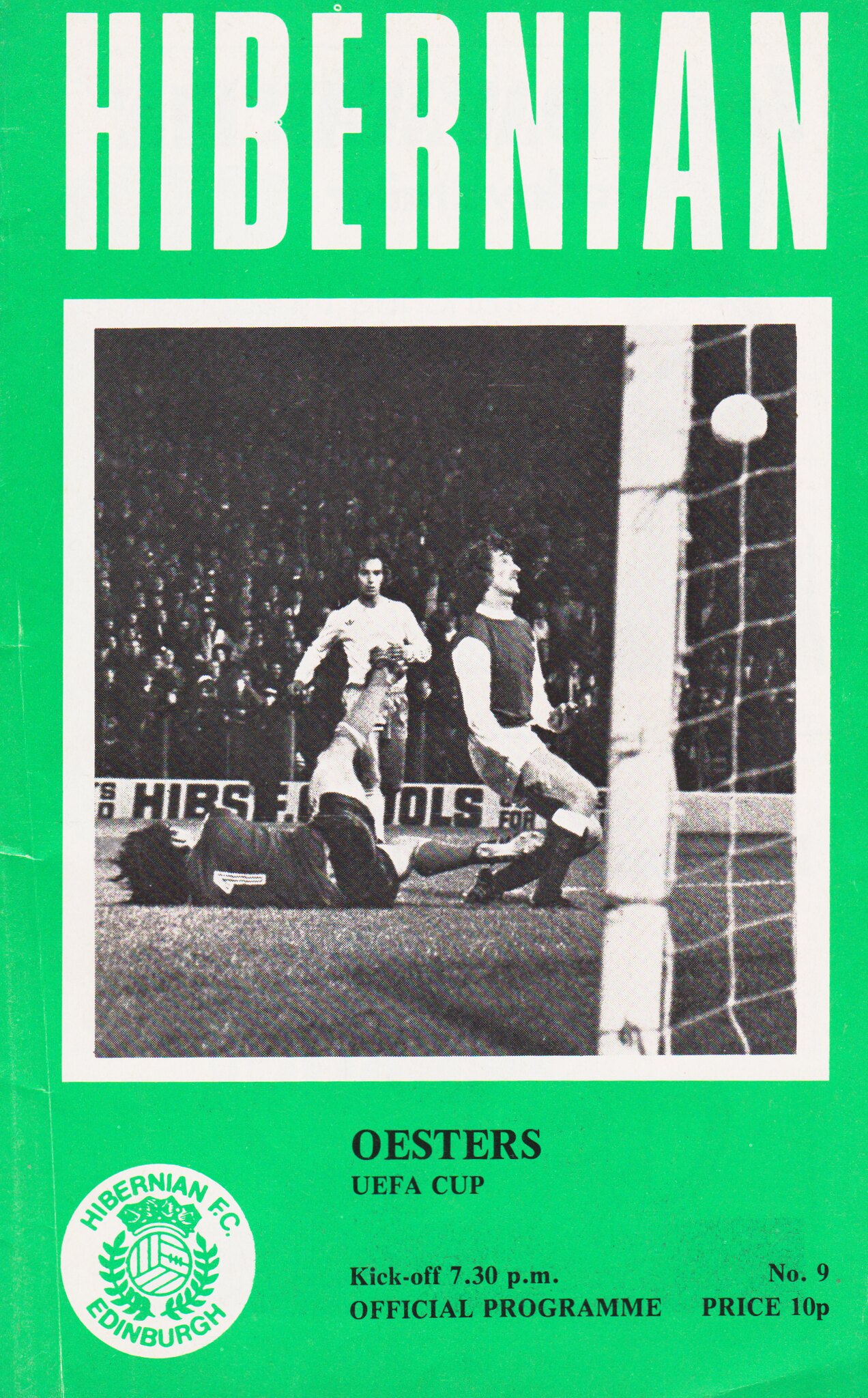The vertical rectangular cover of the program, predominantly green with a limey hue, prominently features the word "Hibernian" at the top in large, bold white letters. Below this, in smaller black text, it reads "Osters" and "UEFA Cup." A black and white action photograph dominates the center of the cover, capturing a dynamic soccer moment near a goal with a white net. The image shows multiple players; one is on the ground with his feet up, another is bent over with knees bent, while the soccer ball hovers in mid-air near them. The players are in white shorts and dark shirts, and it appears one could be a referee. In the lower left corner, there's a white seal featuring "Hibernian FC Edinburgh." Additional text in black at the bottom of the cover includes details such as "kickoff 7.30 p.m.," "number nine," "official program," and "price 10 pence."